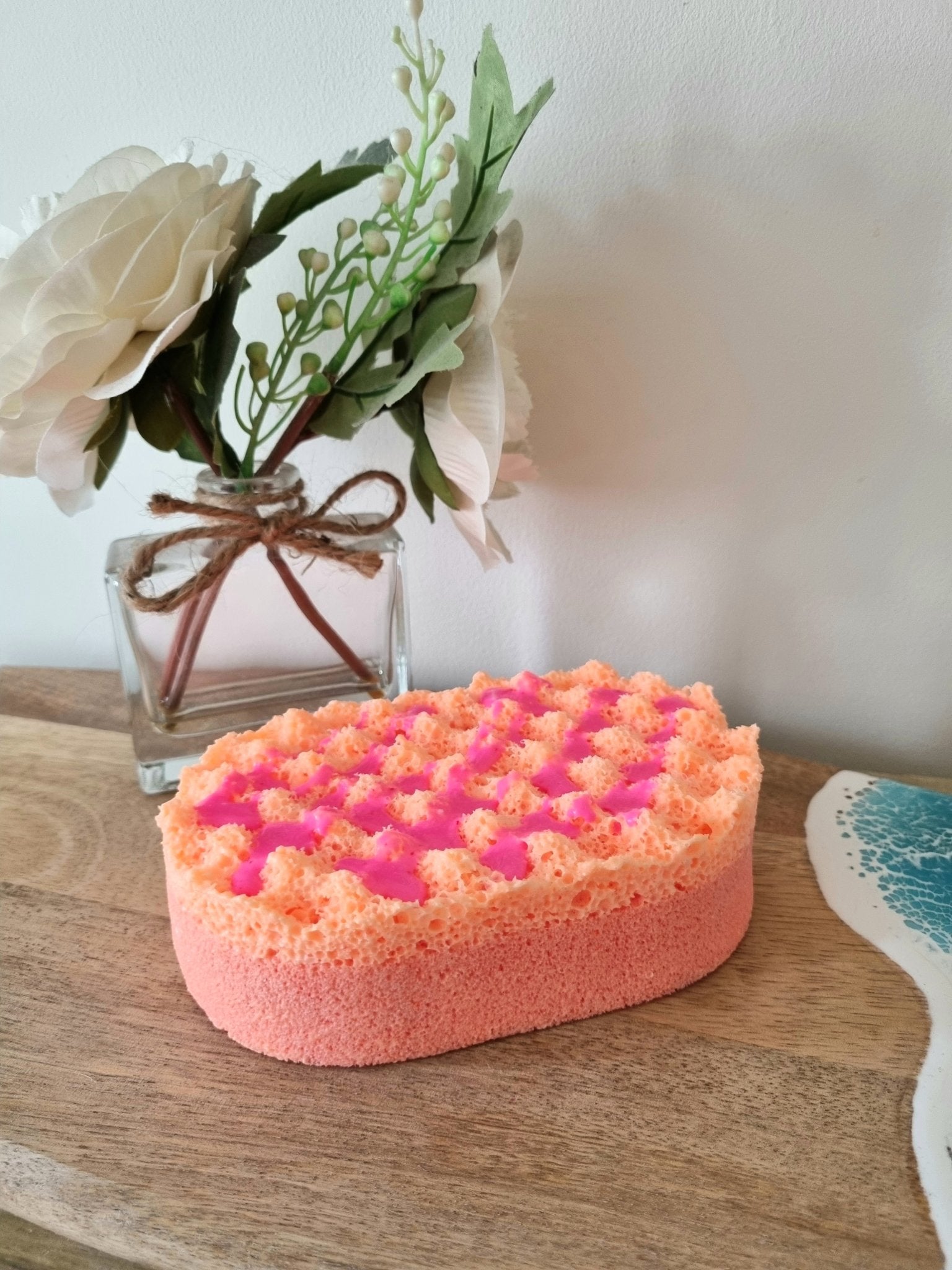In the picture, taken inside, we see a carefully arranged display on a light brown, washed-out wooden board set against the backdrop of a white wall. On the upper left, a rectangular glass vase with a small opening is adorned with a piece of twine tied in a little bow. Nestled in the vase are artificial flowers: a rose with outward-facing petals, possibly made of plastic, and a Lily of the Valley-like bloom curving upwards to the right, surrounded by leaves. On the right-hand side of the board, there is another white flower facing directly to the right. Beside these floral elements, there is an object resembling a sponge, characterized by its uneven surface, pinkish hues, and crown-like points. This sponge has a light orange cream color on the top half and a pink color on the bottom half, with pink diagonal patterns forming diamond shapes. It sits on the wooden board, possibly serving as a decorative piece. Farther to the right, the board also features a small piece of cloth with a white edge and a bit of blue, resembling an ocean wave motif.